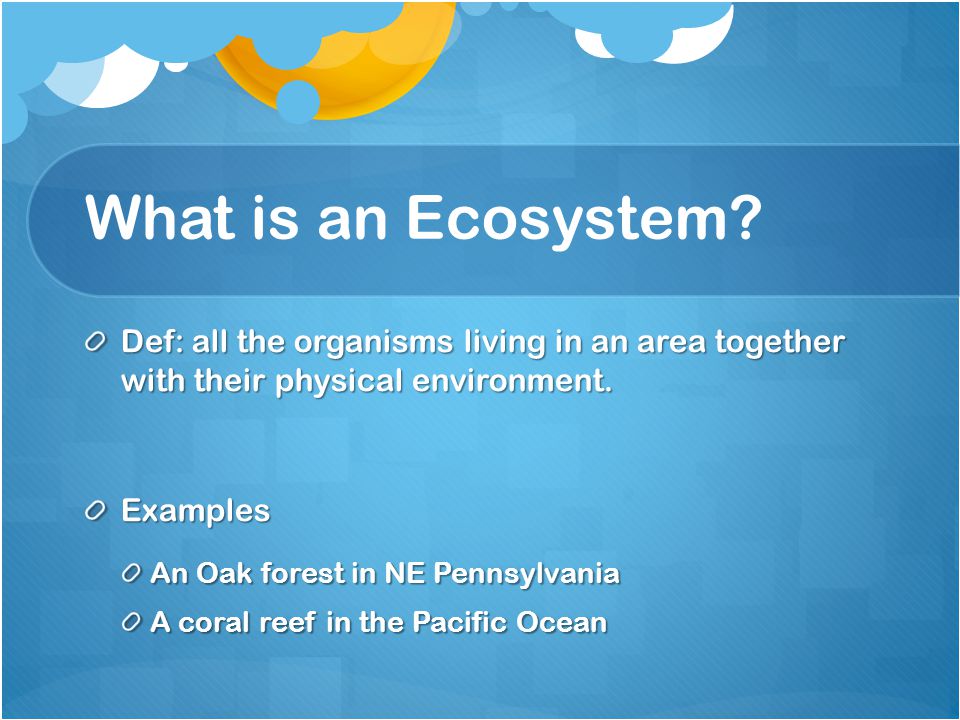The image is an informational slide with a blue background featuring light blue cloud shapes and a depiction of a yellow sun emerging from a white circle at the top. The content is centered around the question "What is an ecosystem?" presented in white letters within a darker blue box for emphasis. Below the title, there is a bullet list, with the first bullet point providing a definition: "All the organisms living in an area together with their physical environment." The second bullet point titled "Examples" lists two specific ecosystems: "an oak forest in Northeast Pennsylvania" and "a coral reef in the Pacific Ocean." The bullet points are indicated by hollow white circles. The slide appears to be part of a larger presentation, designed for educational purposes.